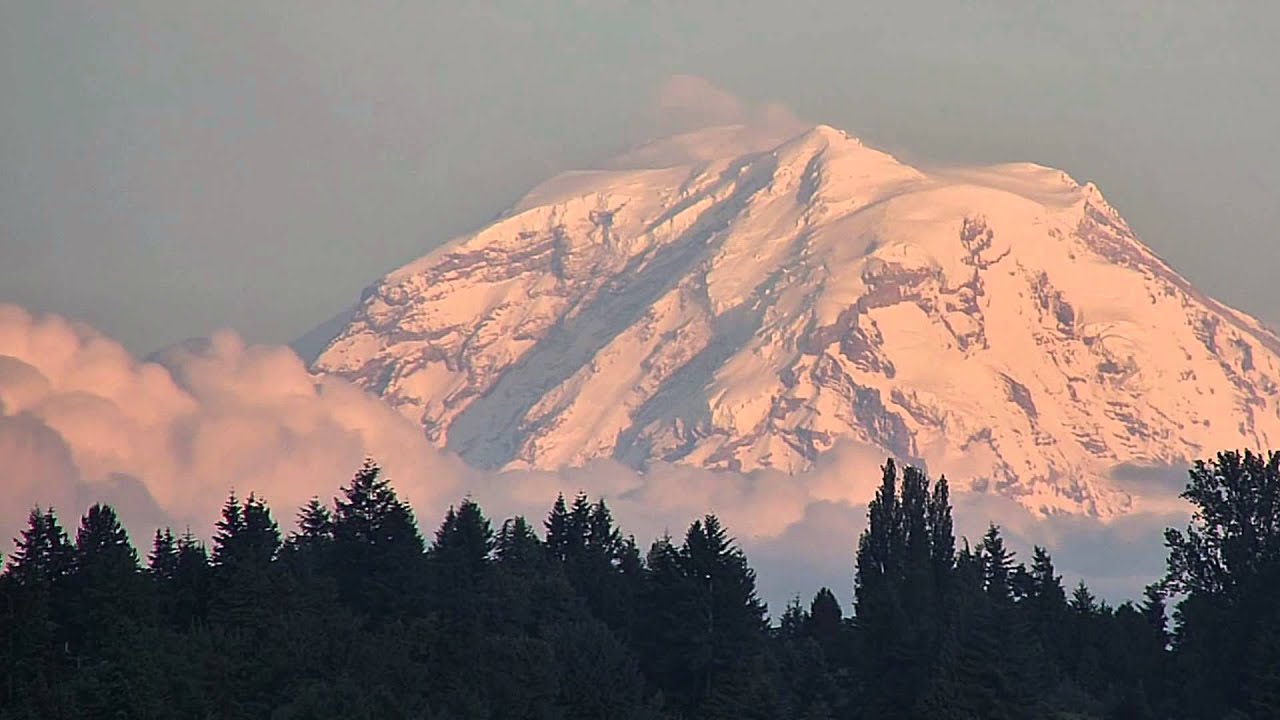The image features a striking landscape dominated by a tall, snow-covered mountain, possibly reminiscent of Mount Hood in Oregon, due to its distinguishable shape. The enormous mountain, adorned with snow and patches of exposed rock, rises majestically at the center and extends towards the right side of the image. Snow trails off the peaks, indicating strong winds, with flurries visibly blowing to the left. Below the mountain, a thick forest of coniferous trees forms a dense tree line that spans the entire bottom fourth of the frame. Above this forest, low-lying clouds roll in, creating a misty transition between the trees and the mountain's base. The sky, a gradient of light blue, white, and gray, completes the scene, suggesting a winter setting possibly during sunrise or sunset, as hinted by the soft light.